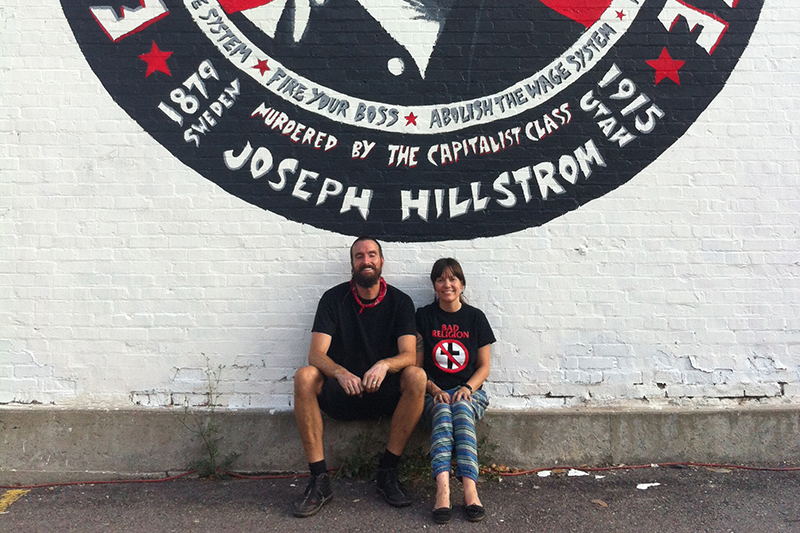A photograph captures two people sitting on a high, gray curb, approximately a foot tall, in front of a white-painted brick wall. The wall is adorned with a large mural, featuring a black circle with white lettering that reads, "Joseph Mills Hillstrom, murdered by the capitalist class, 1915, Utah, 1879, Sweden," surrounded by red stars. Above this are the words, "Fire your boss, abolish the wage system." 

The mural provides a stark contrast to the two individuals seated below. The woman, with her hair pulled back, is dressed in a black t-shirt featuring a no symbol over a cross, and loose blue striped pants paired with black ballet flats. The man beside her sports a black t-shirt, black shorts, black boots, and black socks, accessorized with a red bandana around his neck. He has a beard and mustache. Both appear in good spirits, smiling and seemingly enjoying the moment, despite the serious tone of the mural behind them. The scene takes place in a parking lot with a gray surface, highlighting the contrast between the everyday environment and the striking wall art.